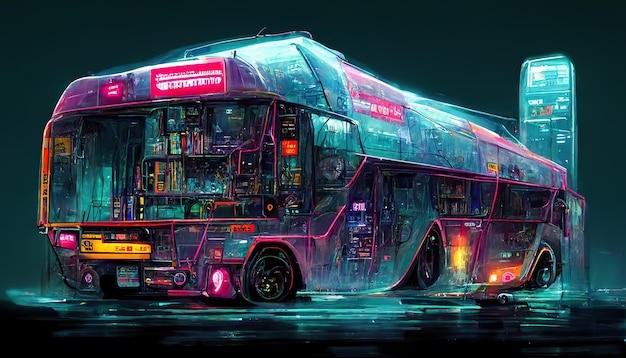This digital art piece features an oversized, neon-colored bus rendered in intricate pixel art style. The bus is extraordinarily large and futuristic, sporting six wheels, with three clearly visible on the left side facing the camera. The vast windshield spans the entire front of the bus, double the size of a typical bus windshield. The exterior is adorned with vibrant, illuminated colors—predominantly aqua teal and neon pink, with accents of purplish red and blue.

A red destination sign, written in an unreadable foreign script, sits above the windshield. The bus also features another pink sign on its upper side, hinting at a possible double-decker structure. Inside the windshield, there's a glimpse of a peculiar interior; shelves filled with books and a small table are visible, though traditional seating appears absent, lending a unique, almost library-like atmosphere.

The backdrop of the image includes a monumental bluish-teal building that evokes a cyberpunk pirate theme. The night sky contributes to the scene's dark ambiance, with the ground below the bus appearing wet and reflecting streaks of teal light, possibly suggestive of water or shiny pavement. The overall aesthetic is one of striking neon colors and futuristic design elements, creating a surreal and captivating visual experience.